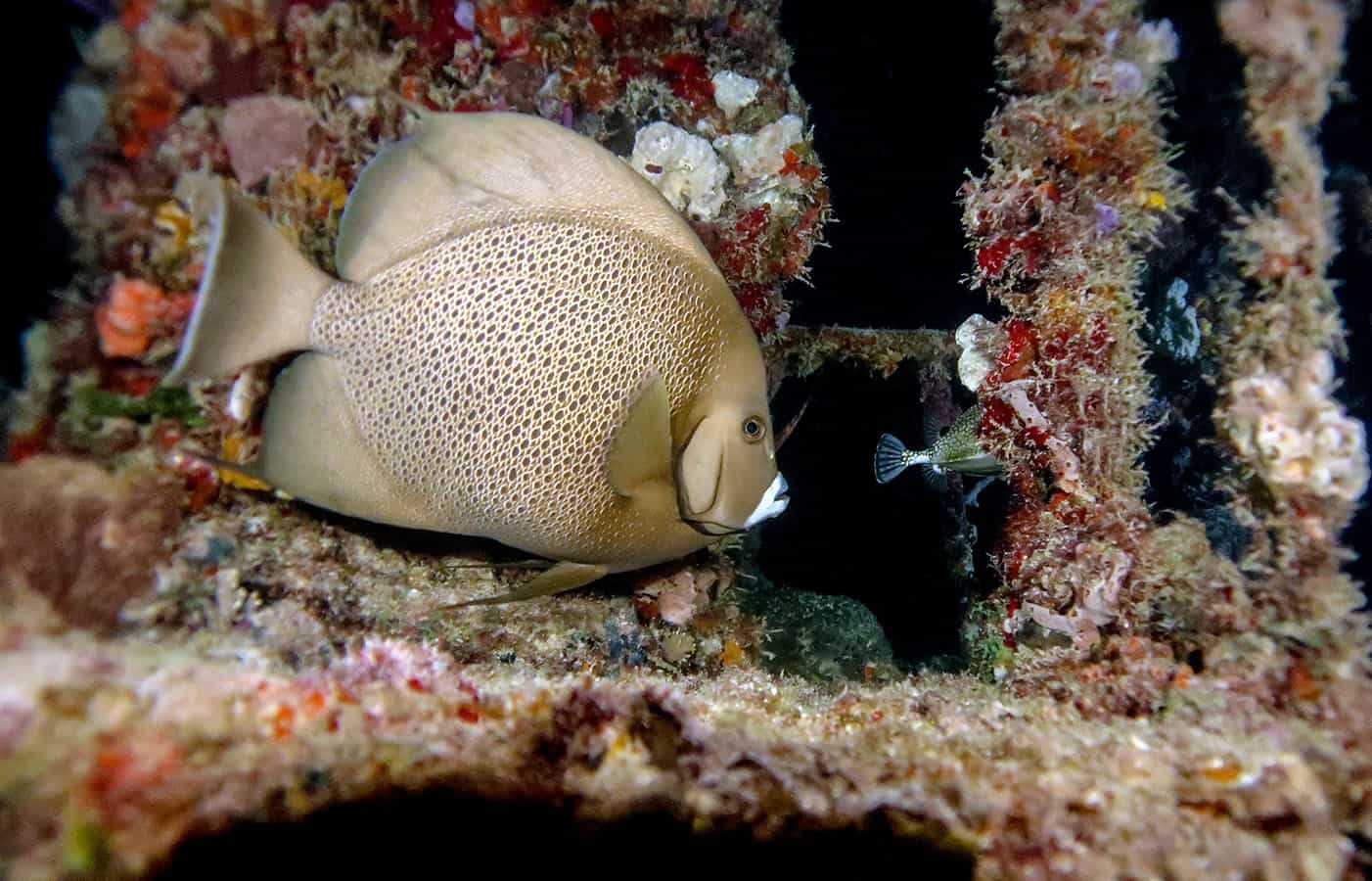This is a detailed and professional underwater photograph capturing a large, fat fish. It features a whitish, light brown body adorned with brown speckled polka dots or tiny dark circles, giving it a scaly appearance. Notable lighter copper skin surrounds these spots, adding texture to its round physique. The fish's mouth area is highlighted with white bits, and its small circular eye is clearly visible at the front.

The backdrop is a strikingly dark, almost perfectly black, water which makes the vivid underwater elements pop. Surrounding the main fish, there are captivating clusters of sea matter, possibly coral or algae, forming beautiful collages. These include a kaleidoscope of colors such as red, pink, orange, yellow, blue, purple, and various shades of brown and white, resembling rainbow-like clumps. 

In addition, there is another smaller fish visible behind the main subject, partly obscured by the coral. This additional fish appears to be green and blue, adding more dimensions to the scene. The entirety of the photo is crisp and in focus, providing a clear and mesmerizing view of this underwater tableau.